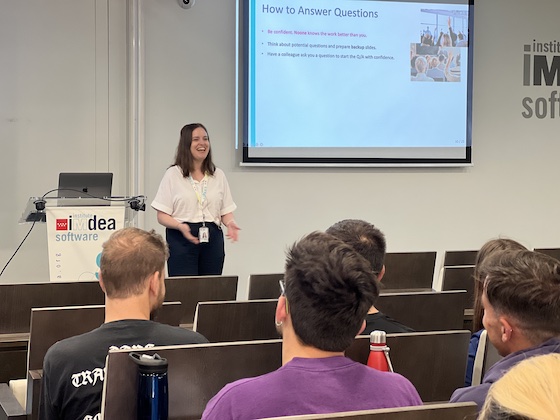In a classroom or presentation room with many empty seats, a woman with shoulder-length brown hair is delivering a lecture to a small audience. She stands next to a white podium with an Apple laptop on it, and the front of the podium reads "I Am DEA Software." The woman, identified by her white-blouse and navy-pants attire in one description, also has a lanyard and badge around her neck as identified by another. She is smiling and gesturing with open palms towards the audience. In front of her, a TV-like display or projector screen shows a slide titled "How to Answer Questions," featuring three bullet points and images of people raising their hands. Five audience members are visible from the back, sitting together in the third and fourth rows. Four of them are men, one is a woman, and they all appear to have light skin. Scattered around them, the rest of the seats remain largely unoccupied.